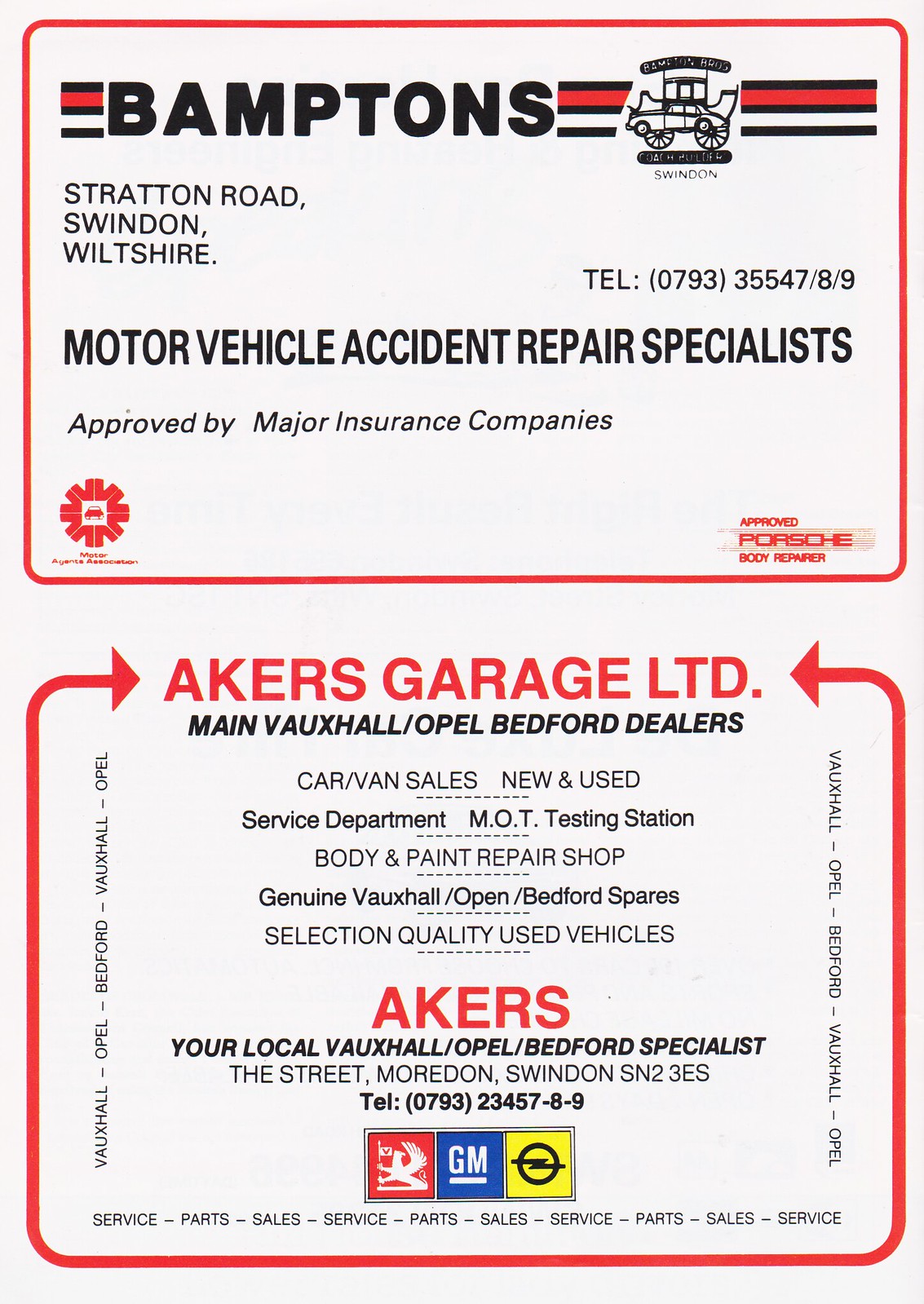The image depicts two business cards placed one on top of the other, both featuring a red-themed design and related to automotive services. The top card is for Bampton's Motor Vehicle Accident Repair Specialists. It prominently displays the company name "Bamptons" in bold capital letters, accompanied by an image of a car. The card provides contact information including an address at Stratton Road, Swindon Wheelchair, and a telephone number (07933 5547-89). Additional details highlight the company's expertise in motor vehicle accident repairs, emphasizing approval by major insurance companies, and specific endorsements like "Approved Porsche Body" in red text, alongside a red star-shaped symbol.

The card beneath it is for Acres Garage Limited, identified as main dealers for Vauxhall, Opel, and Bedford vehicles. The contact address reads The Street, Morton, Swindon, SN2 3S and includes a telephone number (07932 3478-9). It details a wide range of services including car and van sales, both new and used, a service department, MOT testing station, body and paint repair shop, and genuine spare parts for Vauxhall, Opel, and Bedford vehicles. A repeating tagline "Service parts sale service parts sale" borders the card, reinforcing their offerings. The card also features symbols including a bird, a GM logo, and a lightning bolt, set against a yellow background.

Together, these business cards represent two automotive service companies offering comprehensive vehicle repair and sales services in the Swindon area.